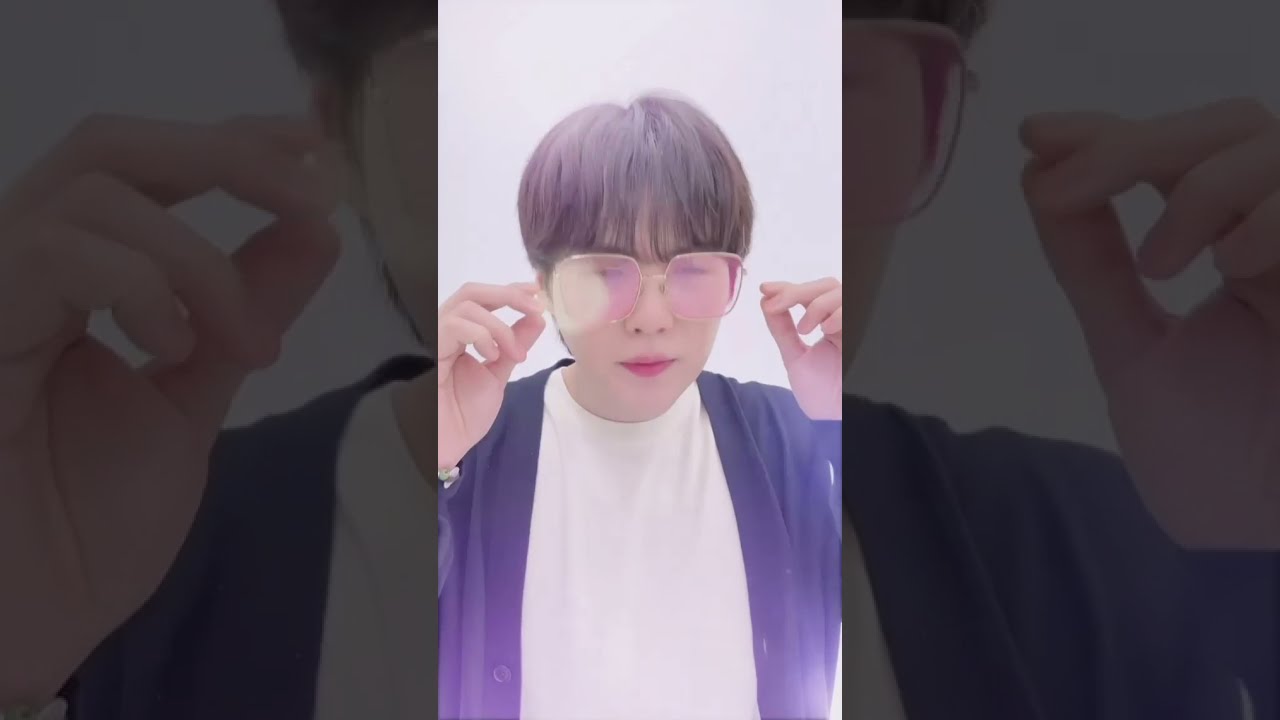The image captures a younger East Asian woman with short, dark hair, sporting long bangs that almost cover her eyebrows, and shorter hair at the back. She is wearing large, square, gold-rimmed glasses with a purplish-pink tint, and her lips are accented with red lipstick. Dressed in a blue buttoned jacket over a white t-shirt, she has her hands raised as if adjusting or just having adjusted her glasses. Her pose suggests a relaxed and casual atmosphere. The background is a light, neutral shade, potentially indicating a minimalist or influencer aesthetic. The central image is set against a mirrored close-up of her face on both the left and right sides, possibly echoing the style of a vertical video, like those found on TikTok. The overall vibe is casual and stylish, with an emphasis on both the fashion elements and the action of the moment captured.